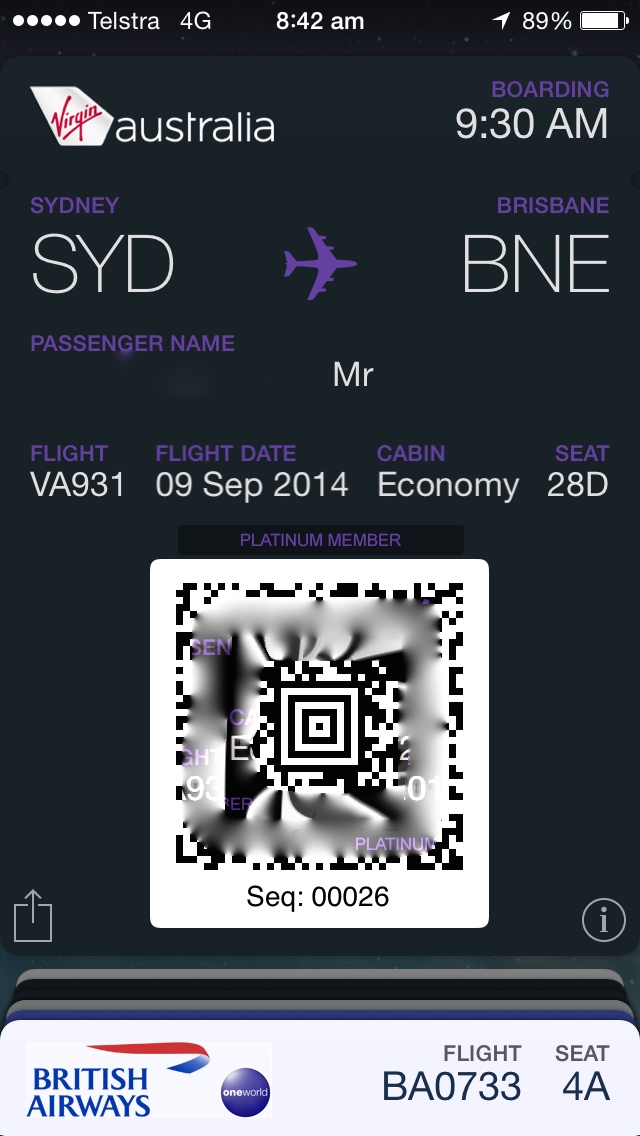This image is a screenshot captured on a cell phone, showcasing a plane ticket or a ticket receipt. At the bottom of the screenshot, there's a QR code that appears as a distorted black and white image. Beneath the QR code, the sequence number "00026" is clearly visible. Directly above the QR code, the title "Platinum Member" is prominently displayed.

Further information is provided above the QR code, including details about the flight:
- **Flight:** VA-931
- **Flight Date:** September 9, 2014
- **Cabin:** Economy
- **Seat:** 28D

At the top section of the ticket, the departure and destination cities are listed, with the departure from Sydney and the destination to Brisbane. Towards the top right corner, the boarding time is specified as 9:30 AM. The airline for this flight is identified as Virgin Australia, as indicated by the Virgin logo next to the word "Australia" in the top left corner.

At the bottom left, there's a small bar that signifies this is associated with British Airways, displaying the flight code "BA0733C4A".